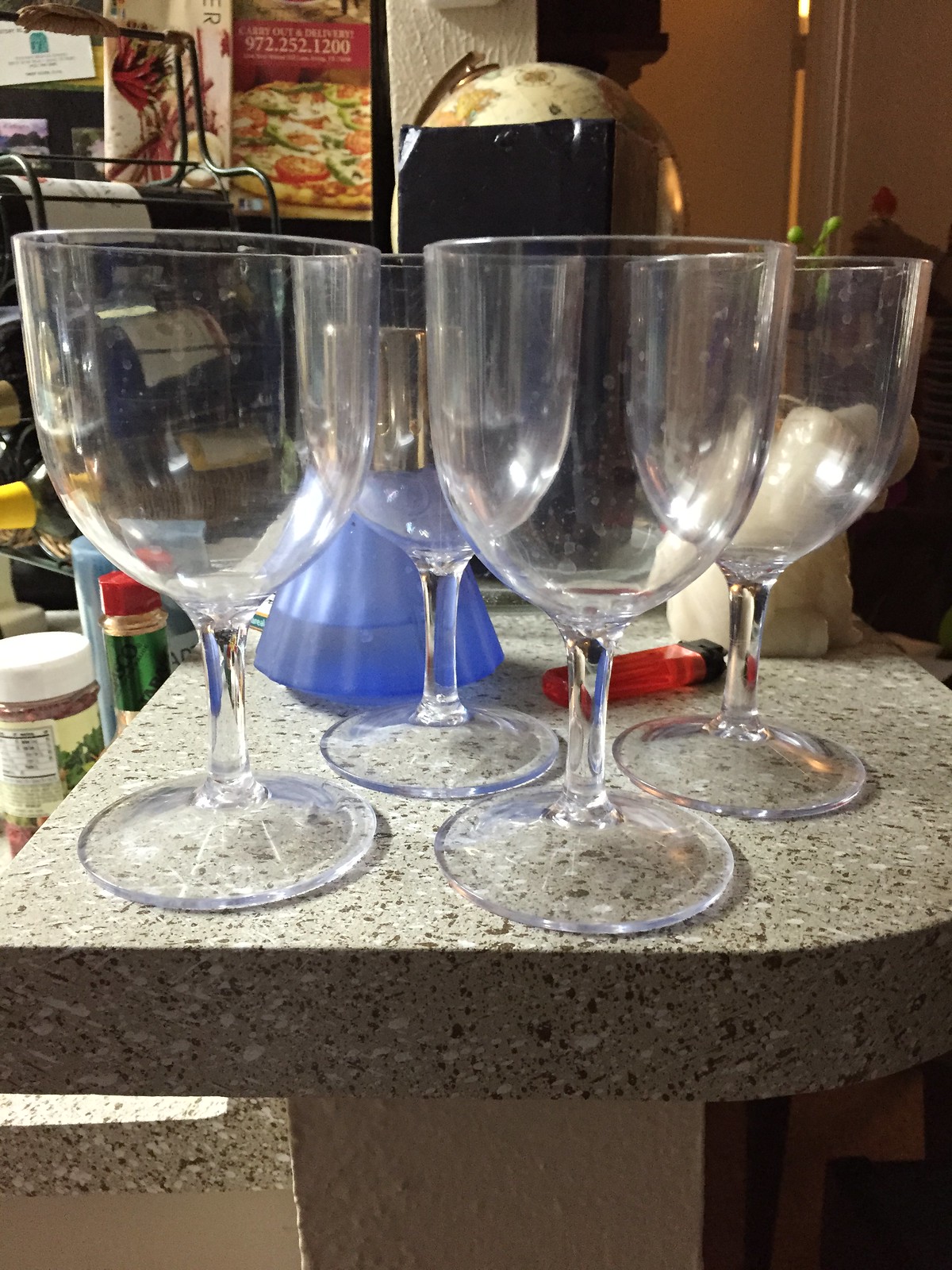This photograph features an interior shot of a kitchen or bar area, taken at a slightly elevated countertop level. The prominent granite countertop, speckled with white and black flecks, spans across the scene. In the foreground, four empty and clean, yet slightly water spotted, wine glasses are arranged in a two-by-two formation, with two in the front and two slightly offset behind. Just beyond these glasses, a clear red disposable lighter rests diagonally on the countertop. Adjacent to the lighter, a blue, fluted bottle with a gold top contains some liquid, adding a splash of color to the setting. A figurine, potentially an elephant or a hippo, is also visible on the countertop, facing away from the camera.

In the background, a variety of culinary elements are dispersed throughout the scene. To the left, a lower counter displays various spice bottles and the partial view of a hot sauce bottle with a red top. Further left, a metal wine rack holds several horizontally aligned wine bottles, positioned below a couple of cookbooks. Above the breakfast bar area to the right, a black object partially obscures a globe. The scene is anchored by a white wall on the far left and a half-open door on the right, adding depth and further context to the bustling kitchen or bar environment.